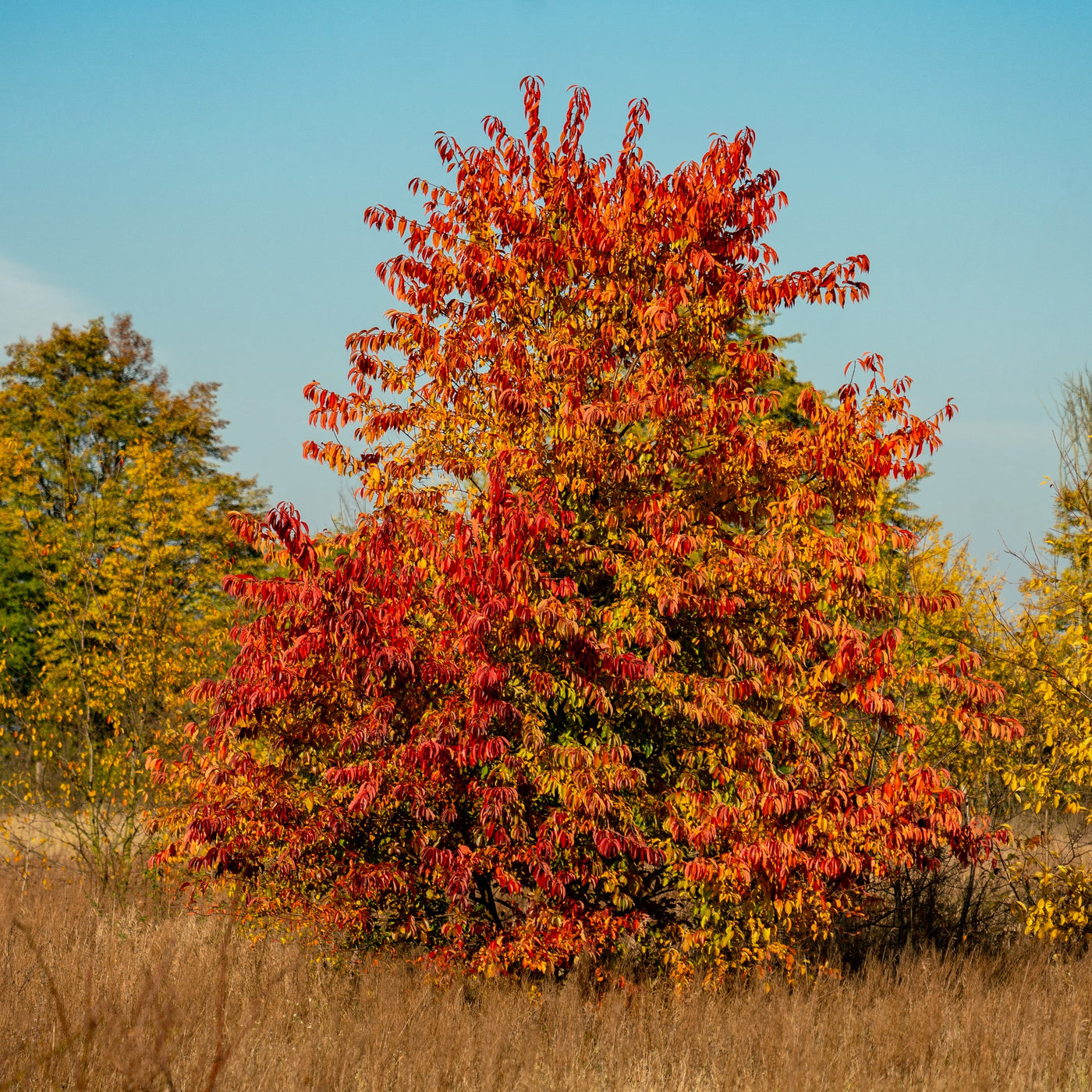The image is a vertical, rectangular photograph capturing a large, prominent tree in the center of a field with tall, brown grass. The tree, strikingly bushy and pear-shaped, is adorned with leaves in various stages of autumn transformation, predominantly red, with about 80% red leaves, and interspersed with yellow and some lingering green leaves near the bottom. This vibrant display marks the onset of fall. In the background on both the left and right sides, there are additional trees, also exhibiting seasonal changes, primarily showcasing yellow leaves. All the trees have branches that extend down to the ground. The scene is bathed in the light of a clear blue sky without a single cloud, enhancing the autumnal atmosphere of the photograph.